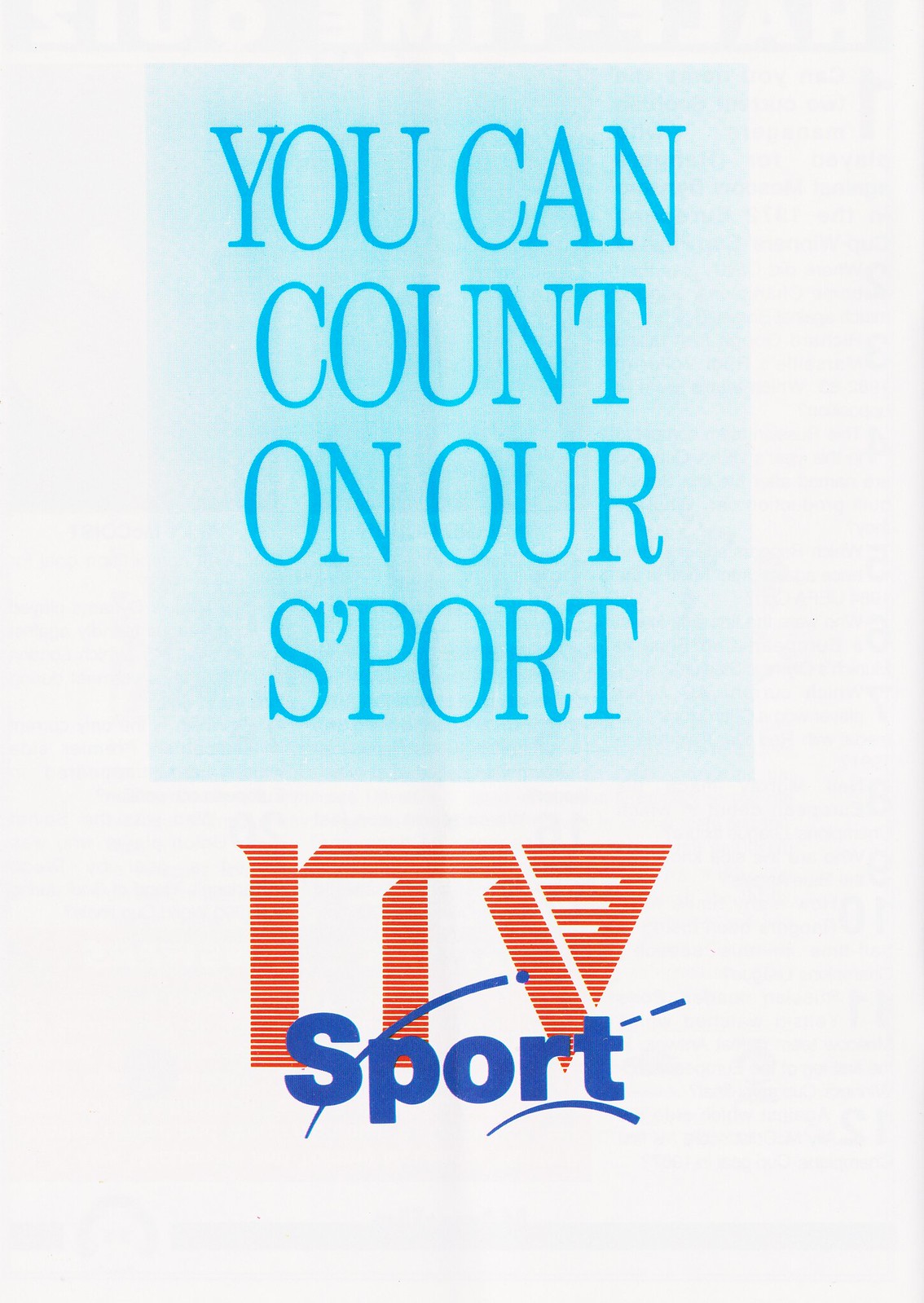The image features a predominantly white background with a rectangular section at the top in a lighter blue. Within this section, bold turquoise text states, "You can count on our sport," with the word "sport" stylized as "S'PORT" to imply "support." Beneath this text is a red, line-stacked symbol forming the letters "ITV," with the "V" uniquely designed with three white diagonal lines. Underneath, the word "sport" appears in bold dark blue, with arcs intersecting the 'S' and 'P' and an additional arc beneath the 'R' and 'T.' The image is portrait-oriented, presenting a clean and professional advertisement, likely for a sports television broadcaster.